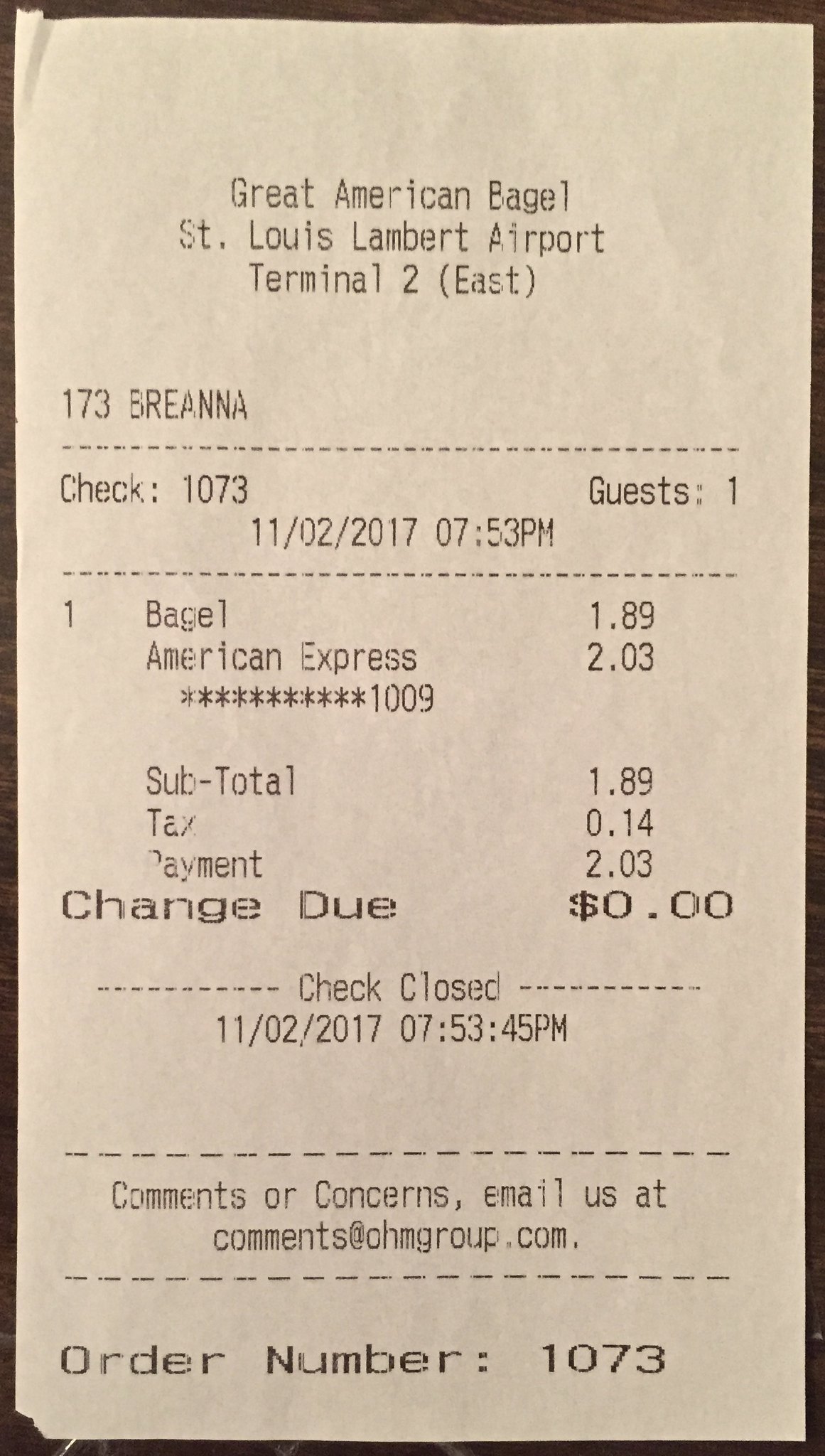The image shows an old, yellowed receipt from The Great American Bagel located at St. Louis Lambert Airport, Terminal 2 East. The receipt, printed in gray or black font on white paper with a slight black border, is dated 11-2-2017 at 7:53 PM. It details an order placed by Brianna, check number 1073, for a single bagel costing $1.89, with an additional tax of 14 cents, making the total amount $2.03. The purchase was paid for using an American Express card ending in 1009. There was no change due. The receipt includes a note for comments or concerns, directing customers to email comment@chmgroup.com, and specifies that the check was closed at the same date and time, 7:53 PM. The receipt appears to be lying on a table, captured in a digital photo with a brown edge visible in the frame.